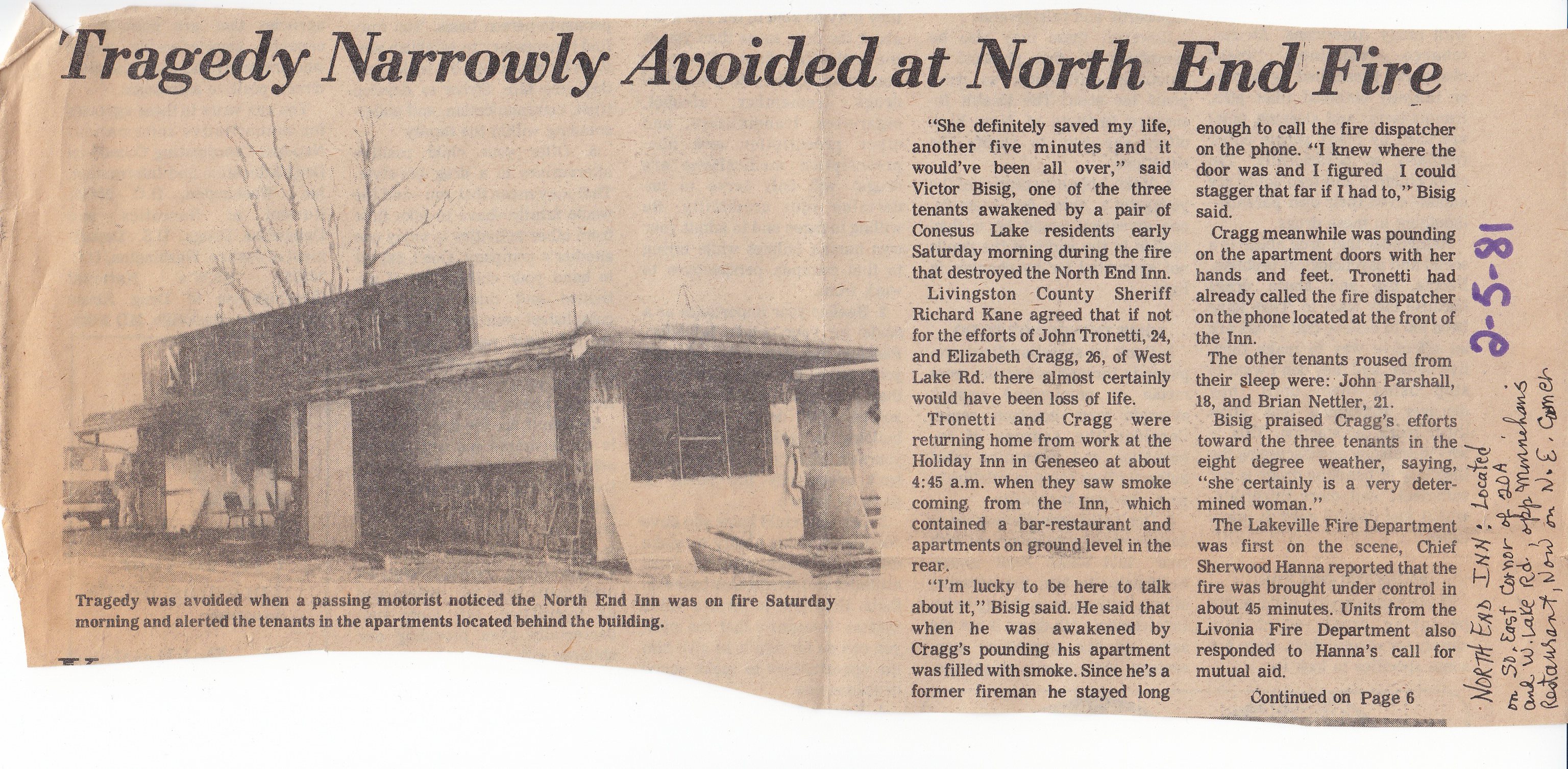The image shows a well-aged, yellowed newspaper cutout with bold black letters at the top reading "Tragedy Narrowly Avoided at North End Fire." On the left, there's a black-and-white photograph of a single-story building, severely burned with a blackened sign above it and various boards scattered on the right. Beneath the photo, a caption reads: "Tragedy was avoided when a passing motorist noticed the North End Inn was on fire Saturday morning and alerted the tenants in the apartments located behind the building."

The right side of the cutout contains two columns of text detailing the incident. The article notes that Victoria Besig, one of the three tenants, credited her survival to the timely warning from John Trenetti and Elizabeth Craig, who were returning home from work at the Holiday Inn in Geniso around 4:45 AM when they saw the smoke. Livingston County Sheriff Richard Kane also acknowledged that their intervention likely prevented loss of life. There is some handwritten text in black ink at the border and the date "2-5-81" written in purple ink.